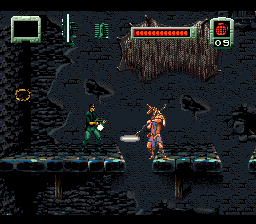An image from a video game showcases a dramatic scene set against a dark, almost completely black background. Despite the dim lighting, two characters are visible, each positioned on their individual platforms that are slightly separated. On the right side of the image, there's a small, armored red player holding a long weapon. The player appears enveloped in the darkness, making it difficult to discern intricate details. On the left, a green character stands out more distinctly; he is uniformly green and holds an illuminated object that lights up part of the scene. At the top of the image, a scoreboard displays "09" in red, accompanied by a nearly filled red bar. Additionally, an amber-colored circle is visible, situated on a section of land that connects to the green character's platform. Despite the overall dark environment, these vivid elements create a sense of tension and immersion within the game.